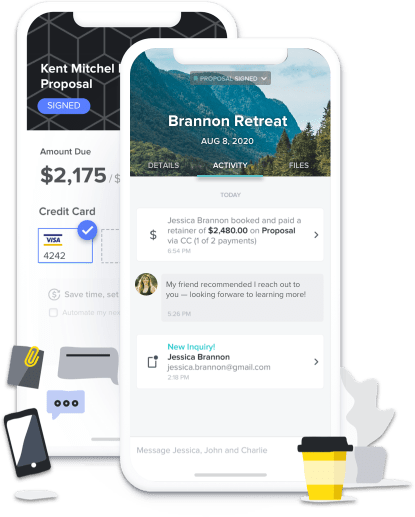The image showcases two iPhone mock-ups, with the front phone partially obscuring the one behind it. Each phone features a screen with a signature display notch. 

On the front phone, the screen is open to an app displaying a page titled "Brandon Retreat, August 8th, 2020." The app is in the "Activity" tab, with two additional tabs labeled "Details" and "Files" visible at the top. The main screen illustrates a list of activities and transactions, starting with a notification indicating that Jessica Brannon booked and paid a retainer of $2,480 via credit card as part of a proposal, marking it as one of two payments.

Below this, there's a message stating, "My friend recommended I reach out to you, looking forward to learning more," followed by another notification about a new inquiry from Jessica Brannon, which prompts the user to click for additional details.

The rear phone's screen appears slightly, displaying content related to payment details for Kent Mitchell's proposal, listed as "Mountain Dew, $2,175." It shows the selection of payment methods, including a credit card ending in 242.